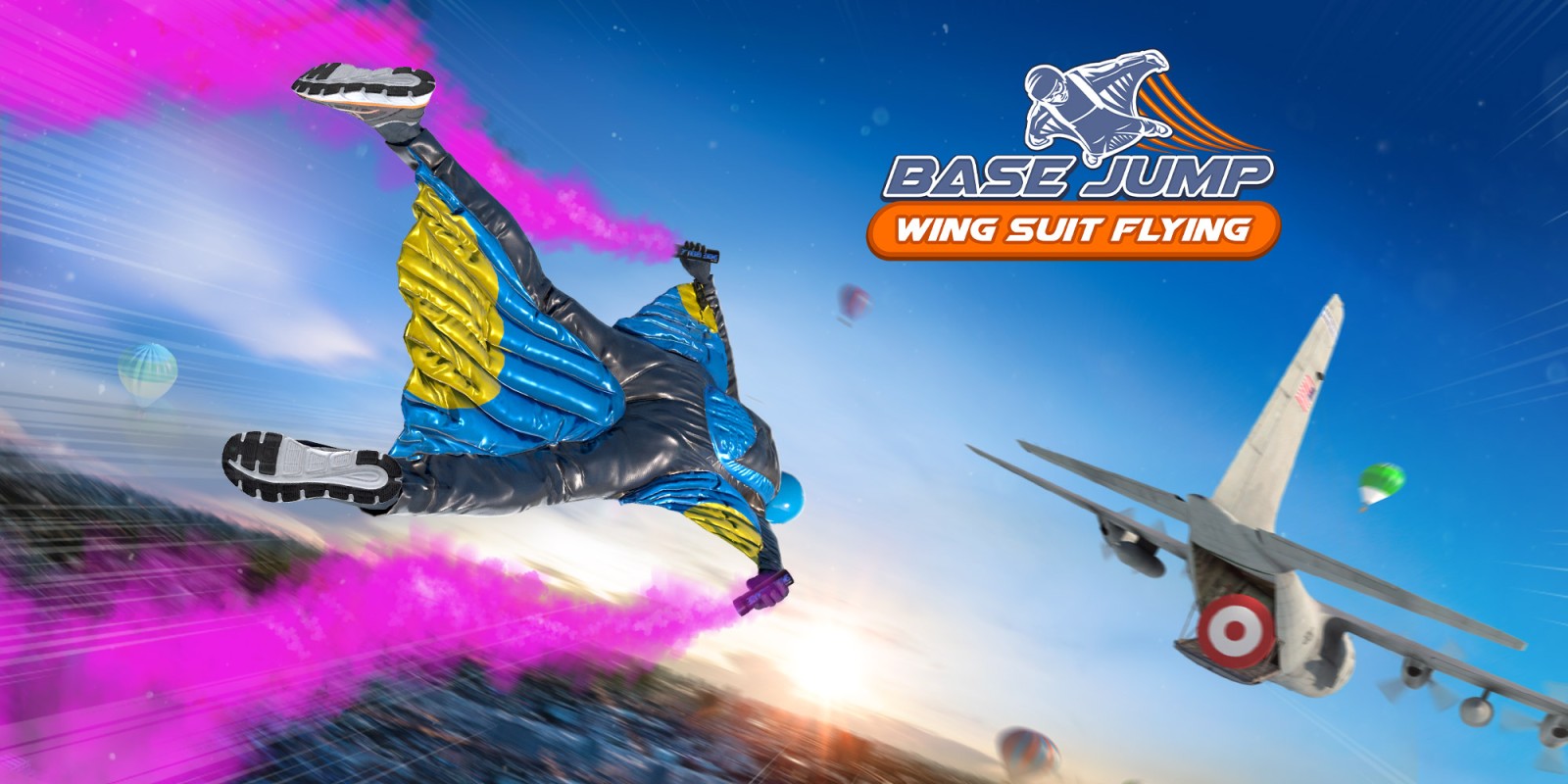The image appears to be a computer-generated advertisement for either a video game or an actual wingsuit flying experience. Dominating the scene is a large transport-style plane with a ramp extending from its tail, situated in the bottom right corner of the image. A distinct red and white bullseye is painted on the ramp, serving as a target. In striking contrast, a person donned in a dynamic wingsuit is depicted soaring towards this bullseye. The wingsuit is primarily blue with darker blue pants, and features wings that are a vibrant cyan teal with yellow semi-circles at the bottom edges. The individual, centered left in the image, has arms outstretched as pink smoke billows from flare canisters held in each hand, giving a palpable sense of motion and direction.

The background reveals a low sunset with a gradient sky transitioning from dark blue in the top right to lighter hues near the horizon. Enhancing the atmospheric depth, four blurred hot air balloons are spotted in the distance. Additionally, there are parachutists visible with red and green parachutes adding to the adventurous ambiance.

Text is strategically placed in the top right corner, stating "Base Jump Wingsuit Flying." The word "Base Jump" is rendered in gray with a white outline, accompanied by an icon of a wingsuited base jumper angled toward the text. Yellow motion lines trail from the jumper, complementing the "Wingsuit Flying" text in white letters on a yellow ribbon beneath "Base Jump."

Overall, the scene captures a thrilling moment of precision and adrenaline, emphasizing the vibrant colors and intricate details of the adventurous flight.